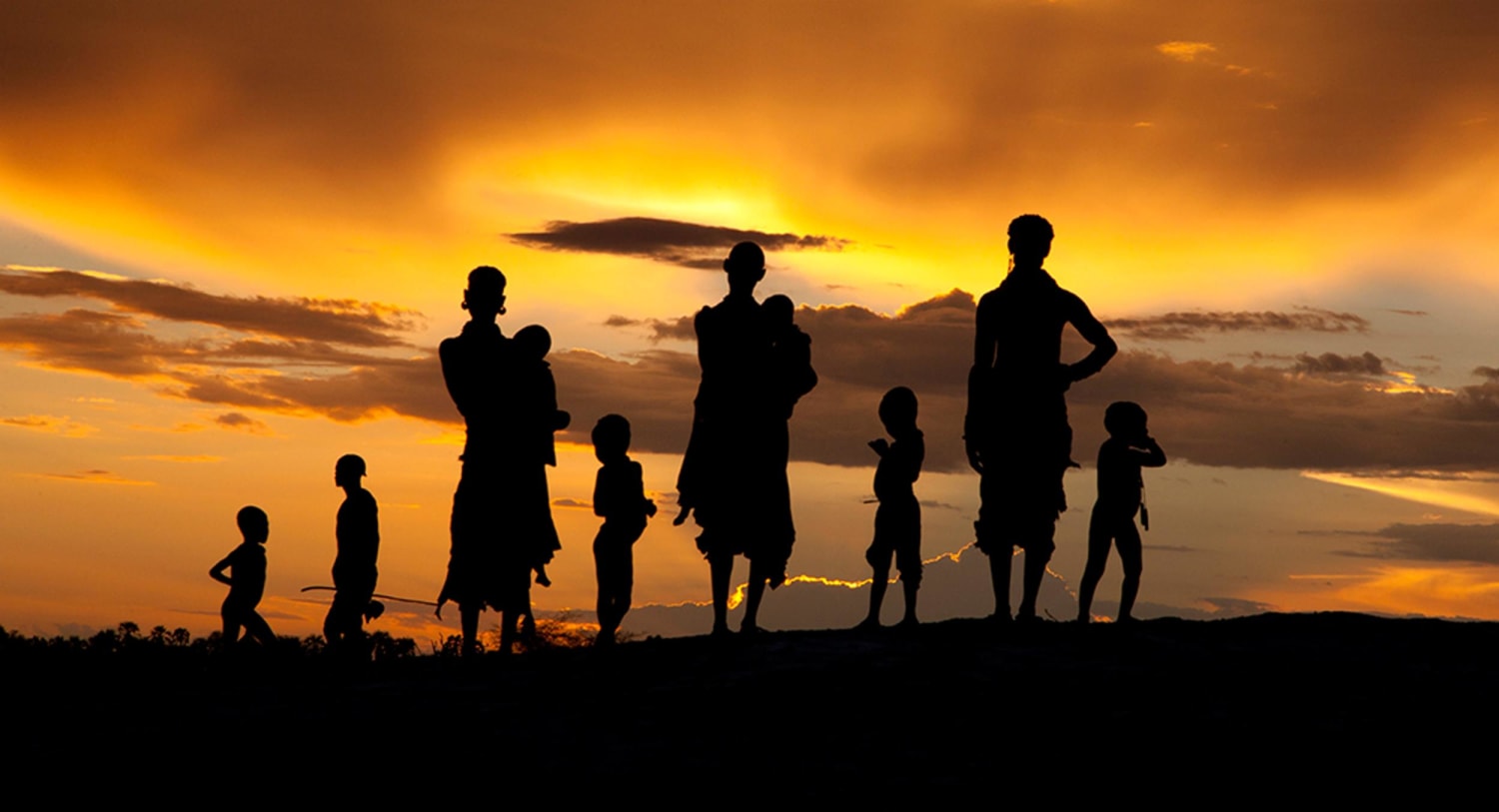In this evocative photograph, a vibrant orange and yellow sunset casts a dramatic glow over an outdoor scene, where the sky transitions to dark gray clouds both on the horizon and up above. The sun is partially obscured by a long, floating cloud in the middle of the sky, which adds depth to the picturesque sunset. Silhouetted against this striking backdrop, eight figures stand on a dark, flat ground, their forms outlined in shadow. Arranged with attention to symmetry, the group consists of three adults and five children. There are two children standing to the left of the leftmost adult, a woman holding a baby. Centrally placed is another child, followed by a second adult woman, also holding a baby. To her right stands another child, and on the far right is the third adult woman, distinguishable by her hand on her hip, standing beside yet another child. These figures are possibly adorned in traditional draped clothing and some carry bows, giving the scene an air of timeless, tribal life. In the distant background, faint silhouettes of trees add an additional layer of depth to this mesmerizing sunset tableau.